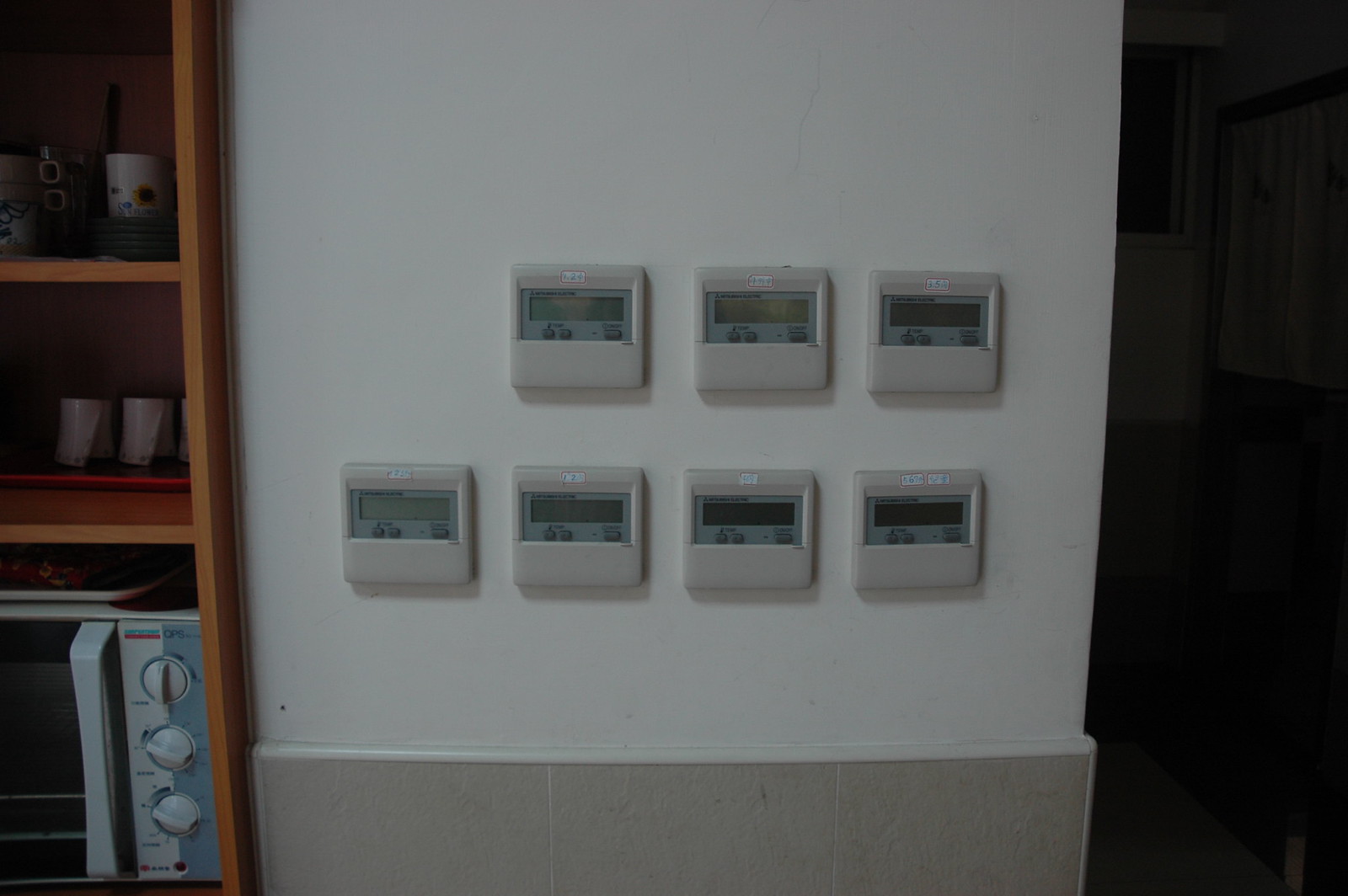The photograph depicts the interior of a home, specifically focusing on a white wall adorned with an unusual array of seven thermostats. The thermostats are arranged in two rows: the top row features three units, while the bottom row consists of four. Beneath the thermostats, there is a section of gray molding that adds a subtle contrast to the wall.

To the left of this wall, the image captures a dark hallway, which is so poorly lit that its details are indiscernible. Adjacent to this, there's a built-in wooden entertainment center or bookshelf. This recessed unit features two shelves stocked with items; the bottom shelf curiously holds a microwave, while the two shelves above display a total of three white candles—two on the middle shelf and one on the top.

Each of the seven thermostats appears identical, characterized by small LCD displays that are not legible from the distance at which the photo is taken. The peculiar quantity and arrangement of thermostats in one room provoke curiosity about their purpose.